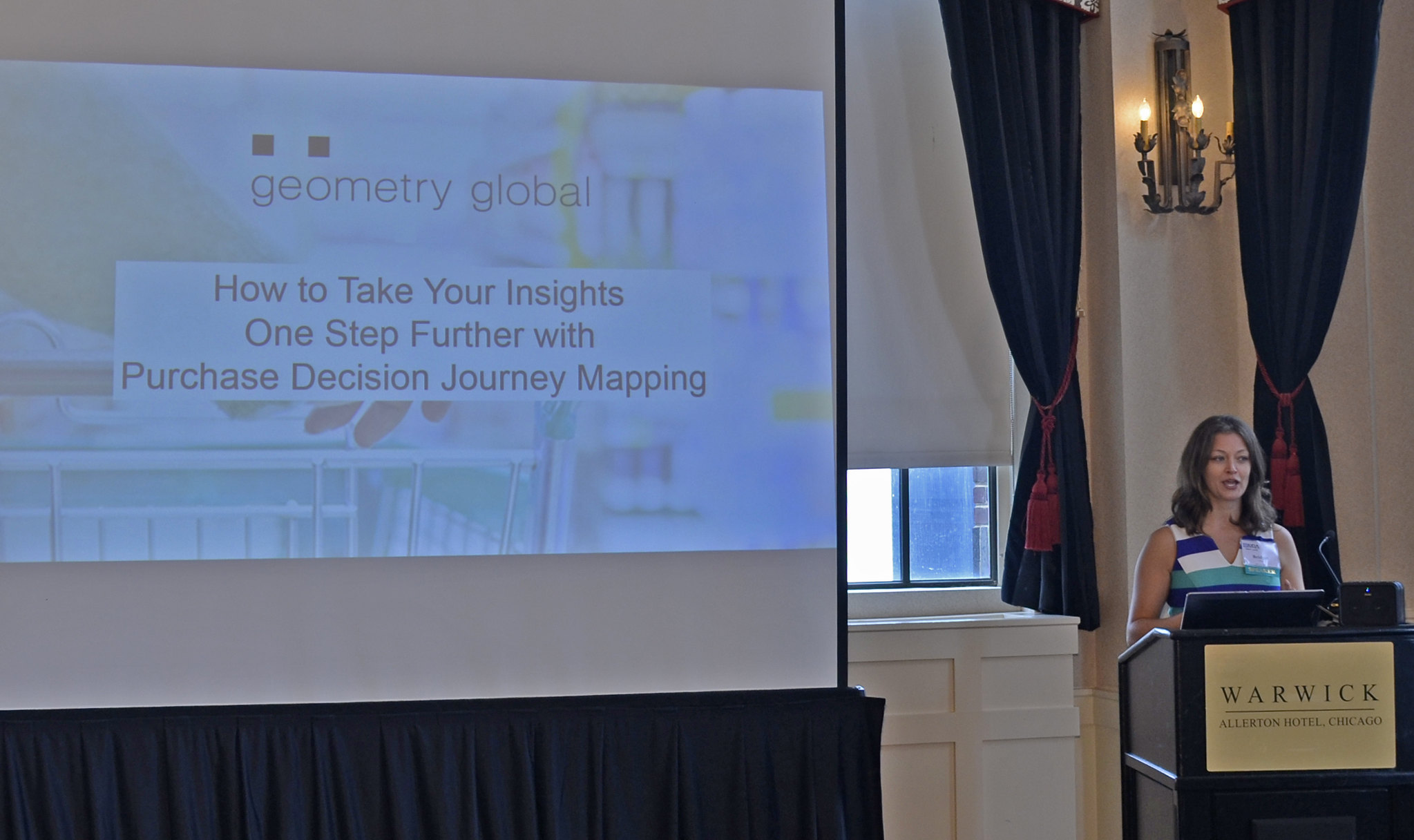In this full-color photograph taken indoors, likely in a convention room at a hotel, a woman stands behind a black wooden podium fitted with a gold plaque that reads "Warwick Allerton Hotel Chicago." The woman, with dark hair, is dressed in a sleeveless V-neck shirt featuring white, dark blue, and turquoise stripes. Positioned to her right, a projection screen displays a slide with the background image of a shopping cart and the text: "Geometry Global, How to Take Your Insights One Step Further with Purchase Decision Journey Mapping." The bottom half of the projection screen is covered by a black curtain. Behind her is a large window framed by black curtains pulled back and tied with red curtain ties, revealing it's daytime. The room is accented by an old-fashioned light fixture above her head, completing the detailed setting of a business conference presentation.